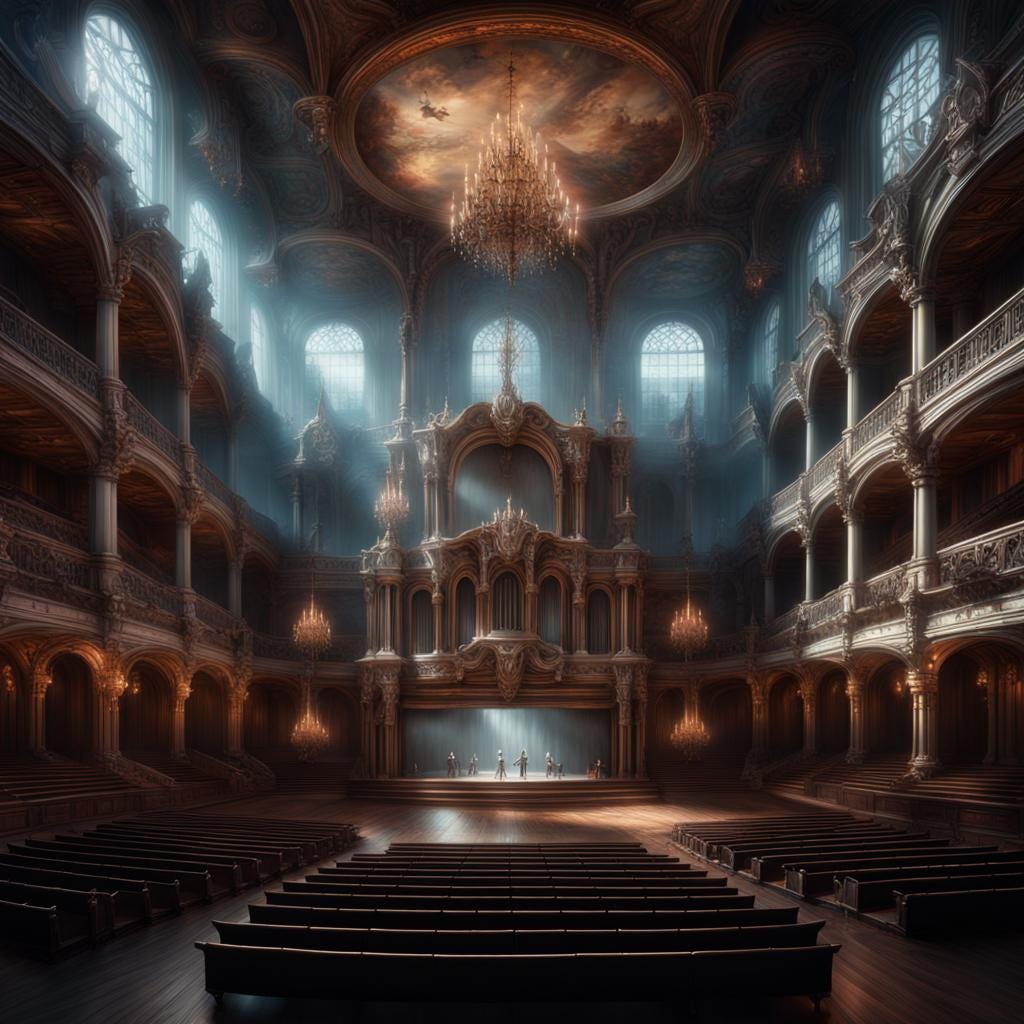A masterful painting captures the essence of an old-fashioned, fantasy theater that exudes both grandeur and mystery. Dominated by ornate wooden carvings and decorative elements, the three-tiered theater features arched windows that bathe the scene in bluish-gray light. The stage, set at the back of three rows of empty benches or pews, is subtly illuminated, hinting at indistinct figures shrouded in dim light. The sides of the theater boast three levels of balconies adorned with intricate wooden railings and posts, providing an elevated view of the stage. Above, a magnificent chandelier with candles hangs from an elaborate medallion depicting orange and yellow clouds or light, adding to the elaborate ambiance. The entire structure, potentially several hundred years old, showcases an array of pillars, arched doorways, and large chandeliers that highlight its historical significance and artistic detail.